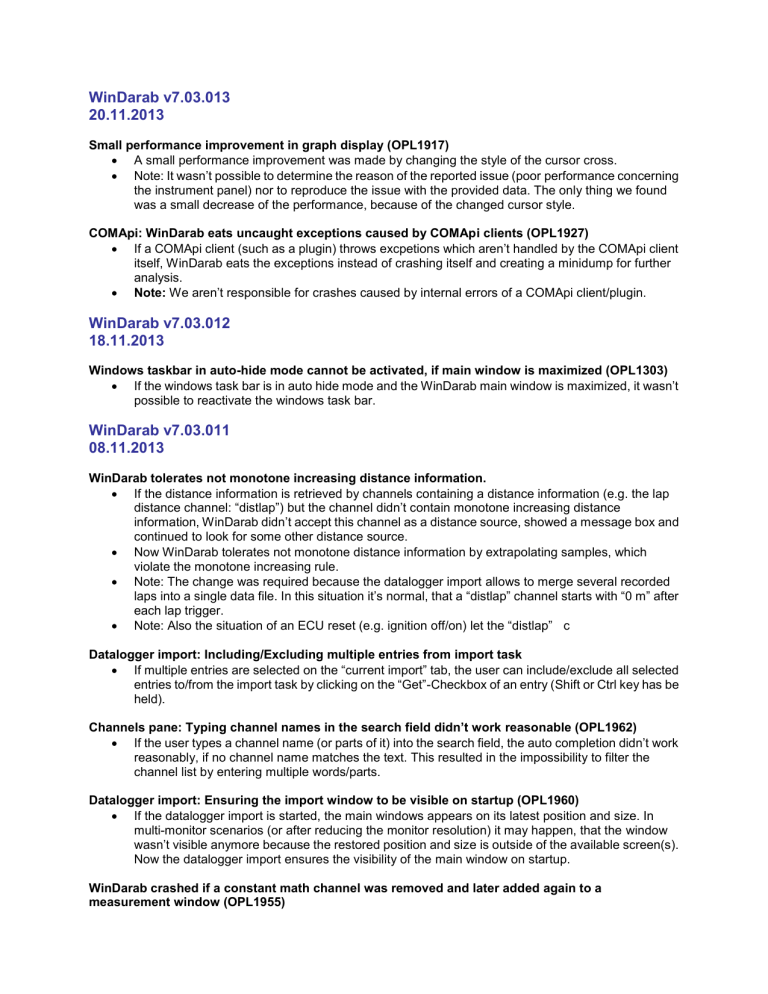A screenshot of the release notes for WinDarab, a software program, is shown. The notes detail three different versions of the software, each with a unique version number and release date. The most recent version, WinDarab 7.03.013, is listed at the top, followed by version 7.03.012, and then version 7.03.011. Each version is released roughly within weeks or days of each other. 

The release notes outline specific changes and improvements made in each update. Version 7.03.011 includes enhanced tolerance for non-monotone increasing distance information in the data logger import and updates to the channels pane. Version 7.03.012 addresses an issue where the Windows taskbar in auto-hide mode could not be activated if the main window was maximized. The latest version, 7.03.013, introduces a small performance improvement in graph display.

The detailed list shows the continuous efforts in refining and enhancing the software's functionality across these sequential updates.